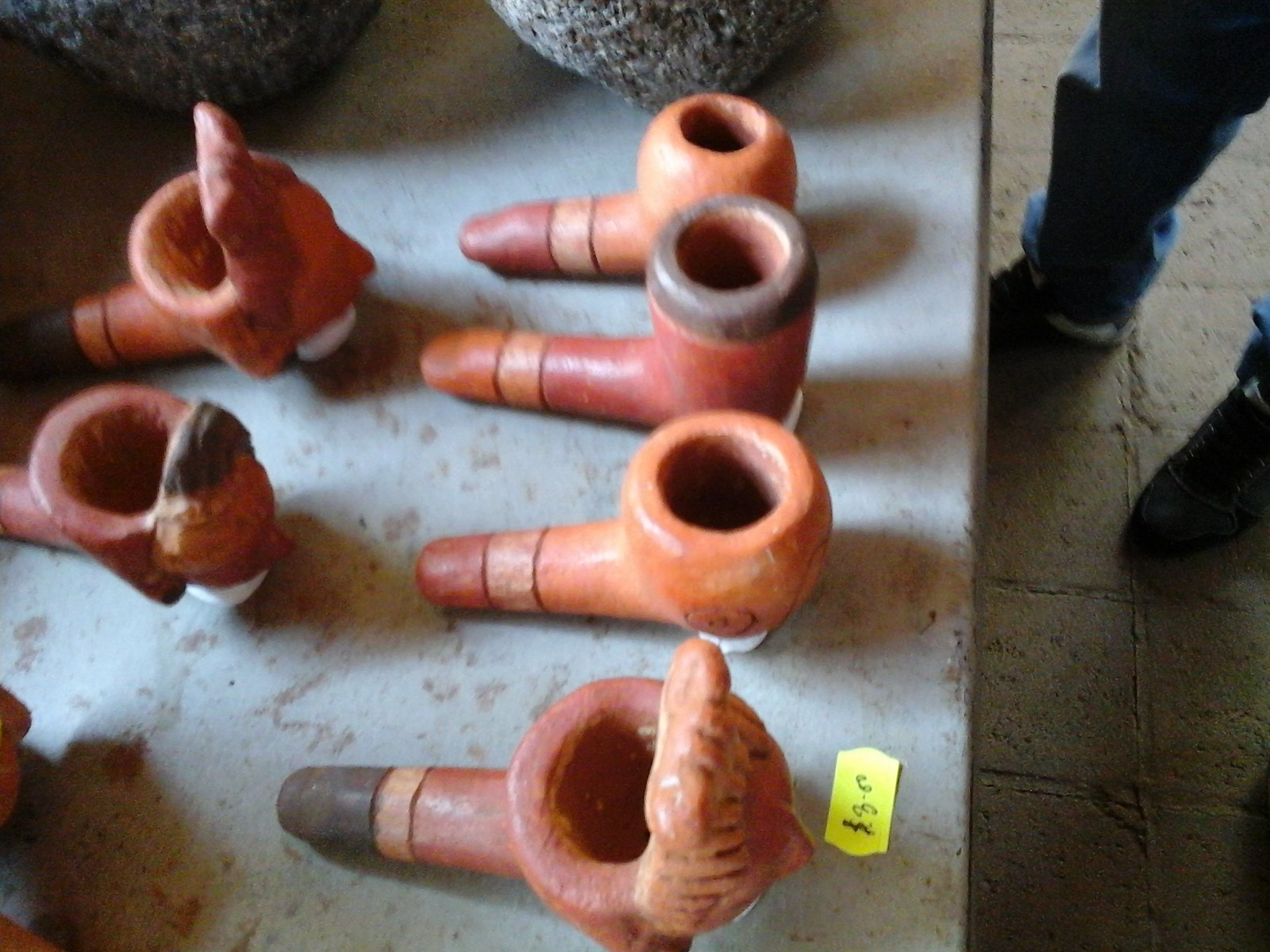This image captures an overhead view of a white marble countertop displaying an assortment of large, clay tobacco pipes. The pipes, primarily orange and clay-colored, are arranged thoughtfully across the table, with the table taking up approximately two-thirds of the left side of the frame and transitioning to a concrete floor on the right. The table is notably dirty, complementing the antiquated appearance of the pipes, which may be part of an archaeological exhibit.

On the right side, intruding into the frame, are the legs of an observer in blue jeans and black shoes, facing left. These legs are visible in the top right corner of the image.

Starting from the upper left corner of the table, a gray boulder partially encroaches into the shot, joined closely by another large boulder to its right. Below these rocks are various pipes. The leftmost pipe is particularly notable for its stylized face and dark black tip, giving it a distinctive, weathered look. Below it, a similar pipe is distinguished by what appears to be brown hair.

Further down, a medium-sized pipe with a dark brown mouthpiece and a lighter brown body sits beneath the rocks. Adjacent to it, another pipe features a dark gray tip, a light brown stripe, and a dark brown body.

An additional pipe near the bottom right resembles the earlier mentioned pipes, maintaining the theme of clay textures and rustic designs. A small yellow price tag indicating "$3.00" is affixed to the table near this final pipe.

Together, these elements paint a comprehensive picture of a collection of beautifully crafted, historic clay pipes displayed on a worn, light-colored surface, juxtaposed against the industrial texture of the concrete floor.